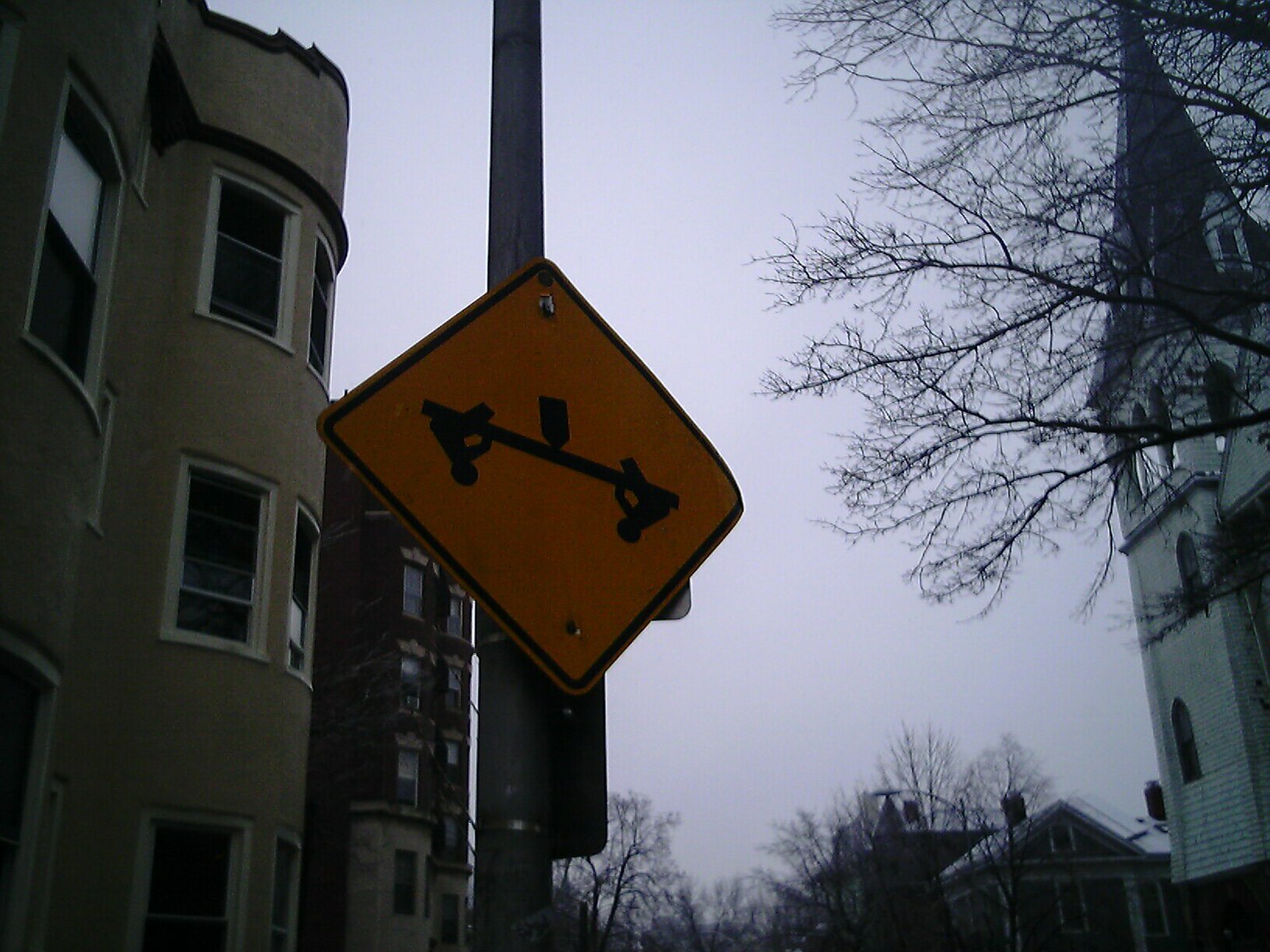In the center of the image, there is a diamond-shaped, yellow warning sign mounted on a stainless steel pole, which has a distinct gray hue. The sign itself depicts two figures appearing to balance on what looks like a horizontal bar. These figures are shown upside down, suggesting some sort of work activity, and at the top center of the sign, there is a shape resembling an arrow pointing upwards. On the left side of the background, a tall building with multiple floors and numerous windows, which could be an apartment complex or condominium, towers into view. Another tall building, dark brown in color with many windows, is visible further in the background. The sky above them is overcast, with thick clouds casting a dim and dark ambiance over the scene, indicating minimal sunlight. The overall atmosphere of the image is rather somber and subdued.